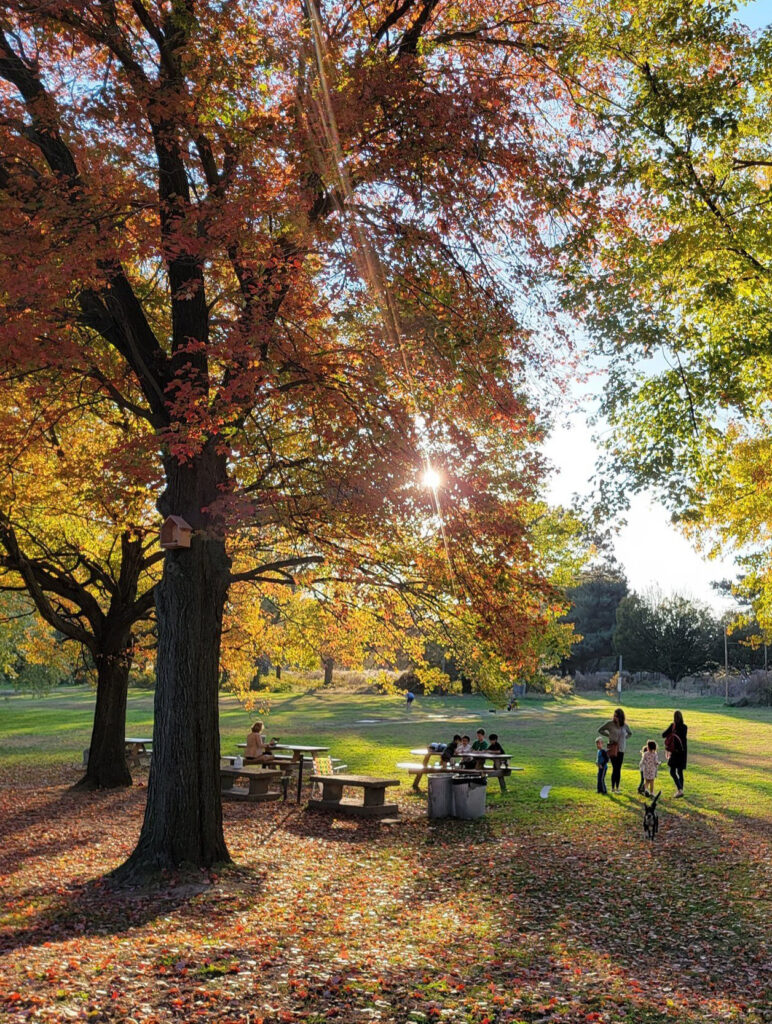This photograph captures a picturesque autumn day at a park. The scene is dominated by two large trees with vibrant leaves in shades of green, orange, red, and yellow, signaling the peak of fall. There are scattered leaves covering the green grass, epitomizing the season’s beauty. A smaller tree is visible in the distance on the left. Beneath the main trees are wooden picnic tables, some accompanied by silver trash cans, where families and groups of children are gathered. One woman, standing with her hands on her hips, watches a child, while another woman sits alone at a table. A highlight of the scene is a small black dog frolicking in the leaves. Adding to the charm, a wooden birdhouse is mounted on the trunk of the largest tree. The sun peeks through the foliage, casting a warm glow across the area and suggesting it's either late afternoon or early evening. The background is dotted with more trees and an expansive grassy area, under a light blue sky. This serene and lively image encapsulates the essence of a leisurely fall day outdoors.